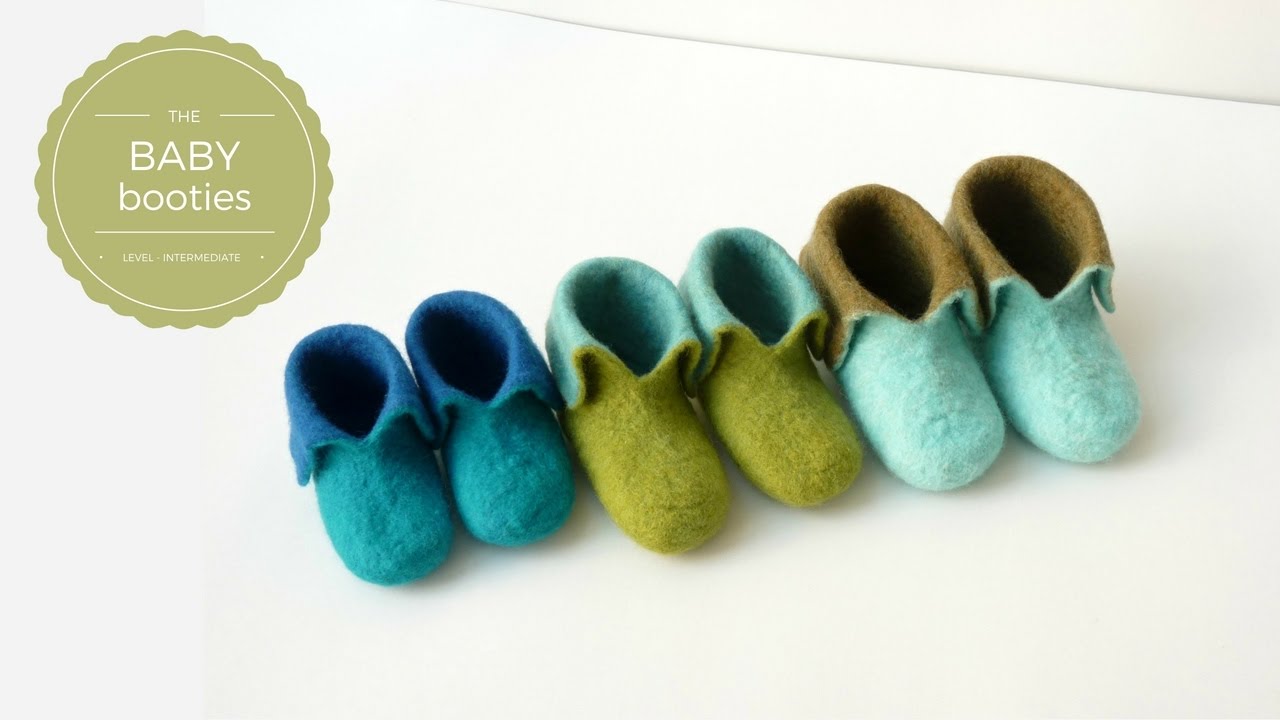The image, resembling a clean advertisement or instructional guide, features three pairs of felt baby booties arranged from left to right on a white backdrop. The smallest pair to the left is dark teal with a dark blue interior, followed by a medium pair in pea green with a light teal interior, matching the exterior of the largest pair to the right, which is light teal with a brown interior. Each bootie has a rounded toe and a turned-down top, suggesting they are slip-on shoes. A beige circular logo with white text in the top left corner reads, "The Baby Booties," followed by "Level - Intermediate," emphasizing the crafting skill required.